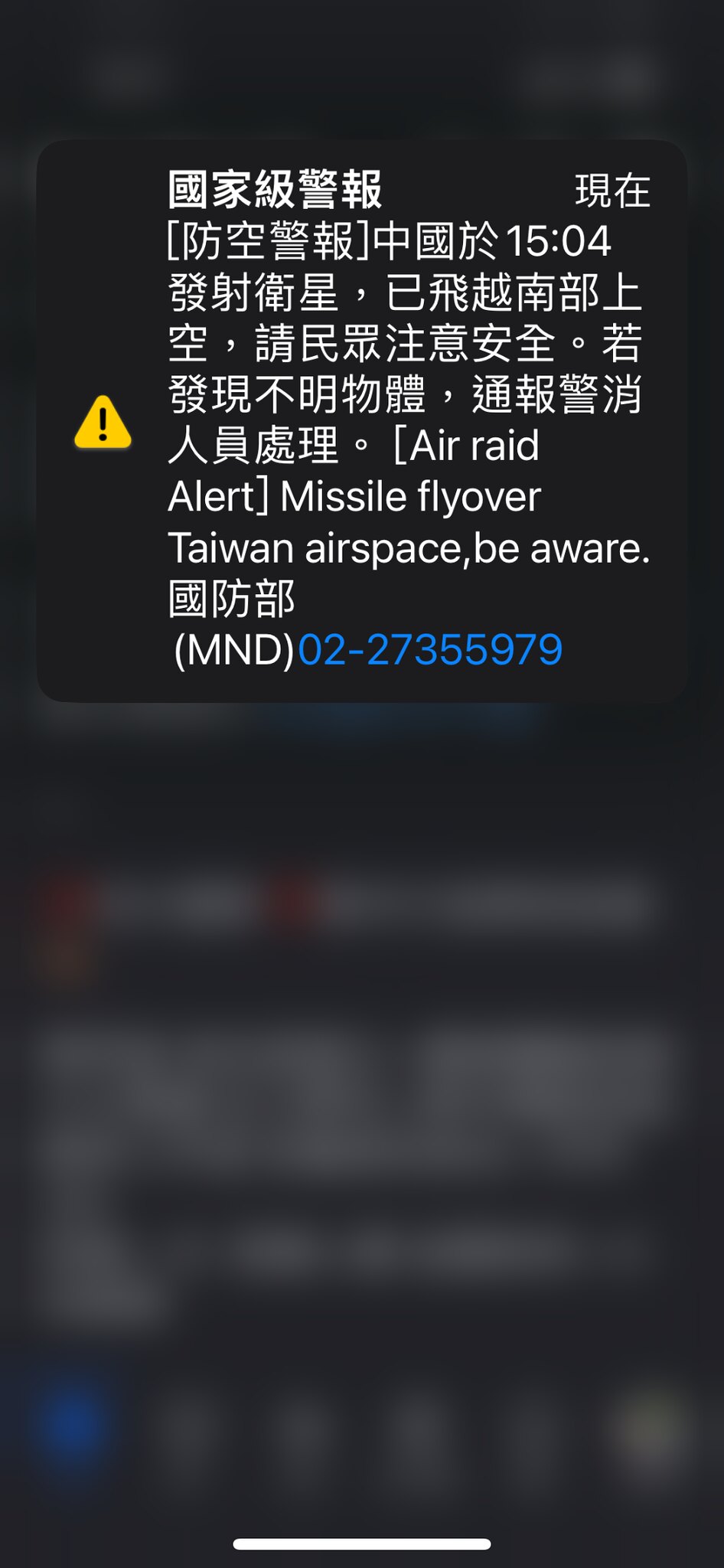The image is a color screenshot, likely from a mobile device or computer screen, with most of it intentionally blurred. The unblurred section shows a yellow triangle with a black exclamation mark inside, indicating a notification box. The visible text includes several lines of Chinese characters, accompanied by the numeral "1504," suggesting the time "3.04 p.m." Below this, more Chinese characters appear, followed by the English phrase "Air Raid Alert. Missile flyover, Taiwan airspace, be aware." Additional Chinese characters ensue, ending with the English acronym "MND" in parentheses. In blue, the text "02-27355979" is displayed. The remaining part of the image is blurred out, emphasizing the urgent bilingual text alert.